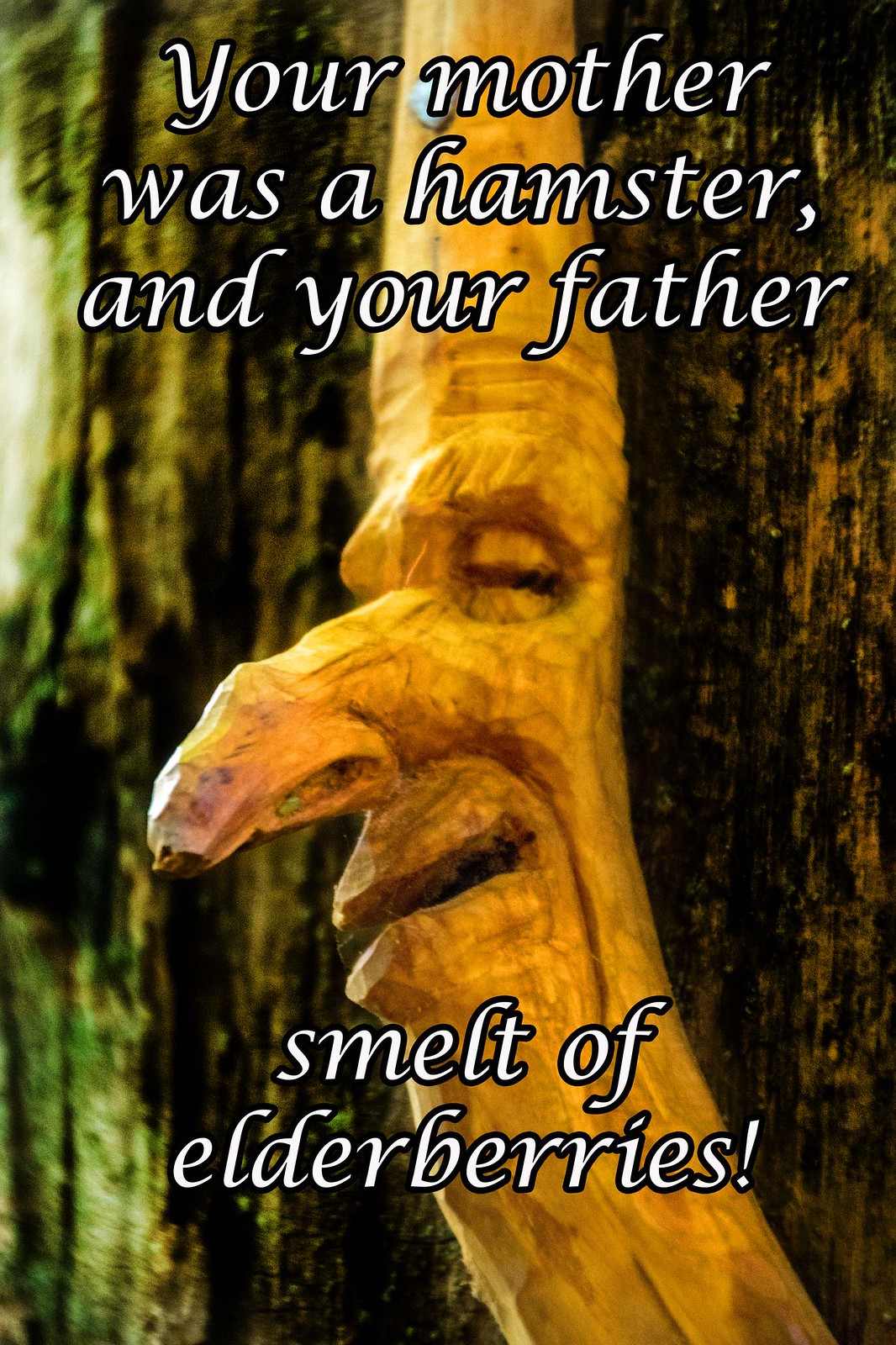The image is a humorous, colored poster featuring a bizarre wooden carving that resembles a humanoid face with an extraordinarily long nose, almost resembling a snake's head at the end. The carving displays distinct eyes, eyebrows, and a twisted open mouth. It appears to be emerging from a worn and dingy tree trunk, evoking a swamp-like atmosphere. The background is filled with the vertical grain of trees. White text, with a slight curve rather than cursive, overlays the image. This text is centered and framed with a black border, quoting a famous insult from the Monty Python movie, "In Search of the Holy Grail": "Your mother was a hamster, and your father smelt of elderberries!" The phrase is split across several lines, with each segment punctuated appropriately, culminating in an exclamation point.